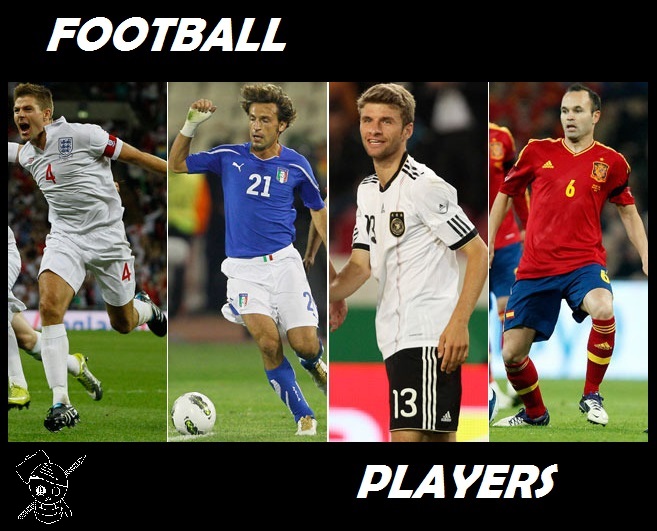The image showcases an intense soccer scene, clearly labeled as "football," reflecting its international context. The backdrop is black, with bold, capitalized white letters in the upper left corner spelling "FOOTBALL." In the bottom left corner, there's a logo depicting a skull, accompanied by the word "PLAYERS" also in large, white font.

Central to the image are four dynamic panels, each highlighting a different soccer player mid-action in distinctive team uniforms. From left to right: 

1. A player in a white jersey adorned with a red number 4, captured in a high-energy moment with his mouth open and legs off the ground.
2. Another in a blue jersey with a white number 21 and matching white shorts, poised to kick a ball positioned in front of him.
3. A third player sporting a white jersey with black detailing, black shorts, and a number 13 on his shorts.
4. Lastly, a player in a red jersey featuring a yellow number 6, paired with blue shorts.

Each athlete is equipped with cleats and shin guards, emphasizing their readiness for the game. The vivid colors—ranging from red and blue to shades of white, black, and green—contribute to the vibrant, competitive atmosphere of the sports arena setting. The players’ positions are centrally aligned between the words “FOOTBALL” and “PLAYERS,” making them the focal point of the image.